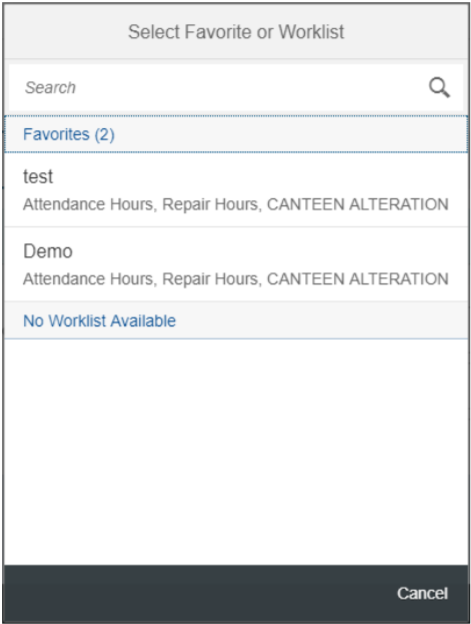This image shows a section of a larger webpage or application interface. At the top of the interface, there is a search bar set against a white background with black text, allowing users to search through the webpage or application. Below the search bar, there are two categories under a tab labeled "Favorites," indicating that there are two bookmarked or frequently accessed items. 

The two listed items are placeholders, one labeled "test" and the other labeled "demo," likely illustrating an ongoing construction or development status. Each item has associated details listed beneath, including "attendance hours," "repair hours," and "canteen alteration," although the exact meanings of these terms are ambiguous within this context. Additionally, below these categories, there is a message stating "No work list available," suggesting that no specific tasks or projects have been assigned yet.

At the bottom right corner of the interface, there is a "Cancel" button for user actions. The background of the entire page is predominantly white, but some sections feature a light gray background, adding subtle contrast. Collapsible and expandable sections within the interface are highlighted with blue font for easy identification. Overall, the interface appears to be part of a management or organizational tool, possibly related to tracking work hours and project statuses.